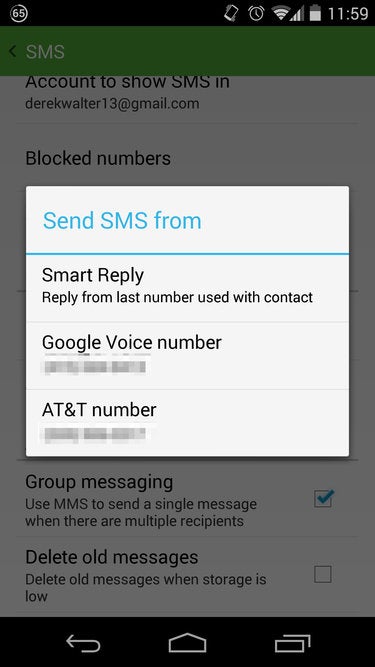The image captures a phone screen displaying the SMS settings page. The background is muted with a gray overtone, highlighting the white section where critical information is presented. At the top of this section, there is the prompt "Send SMS from" in teal color, separated by a line from the next segment labeled "Smart Reply." This segment includes the instruction "Reply from last number used with contact," followed by another faint gray line.

Next, the "Google Voice Number" section appears, with a blurred phone number for privacy. Beneath this, another faint gray line delineates the "AT&T Number" section, where the number is also blurred and smudged to ensure privacy.

In the background at the top of the screen, a green rectangle prominently displays "SMS" in capital letters. This is followed by "Account to show SMS in," with black numbers listed in this section. Further below, there are options for "Group messaging" and "Delete old messages." The overall design is functional, with a clear separation between sections and thoughtful attention to privacy.